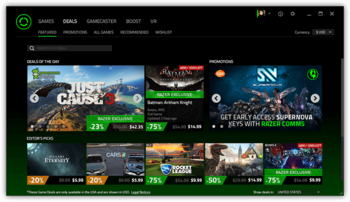This screenshot showcases the interface of a PC gaming website, displayed on a dark-themed background that transitions from black to dark green. Prominent navigation buttons are visible, offering users access to various sections such as available games, special deals, and a feature called GameCaster. Below these navigation options, several advertisements are prominently displayed, highlighting different games available for purchase. Featured games include titles such as "Just Cause" and "Supernova," each accompanied by captivating images from the respective games. The layout is designed to provide users with clear pathways to explore and buy their favorite games efficiently.